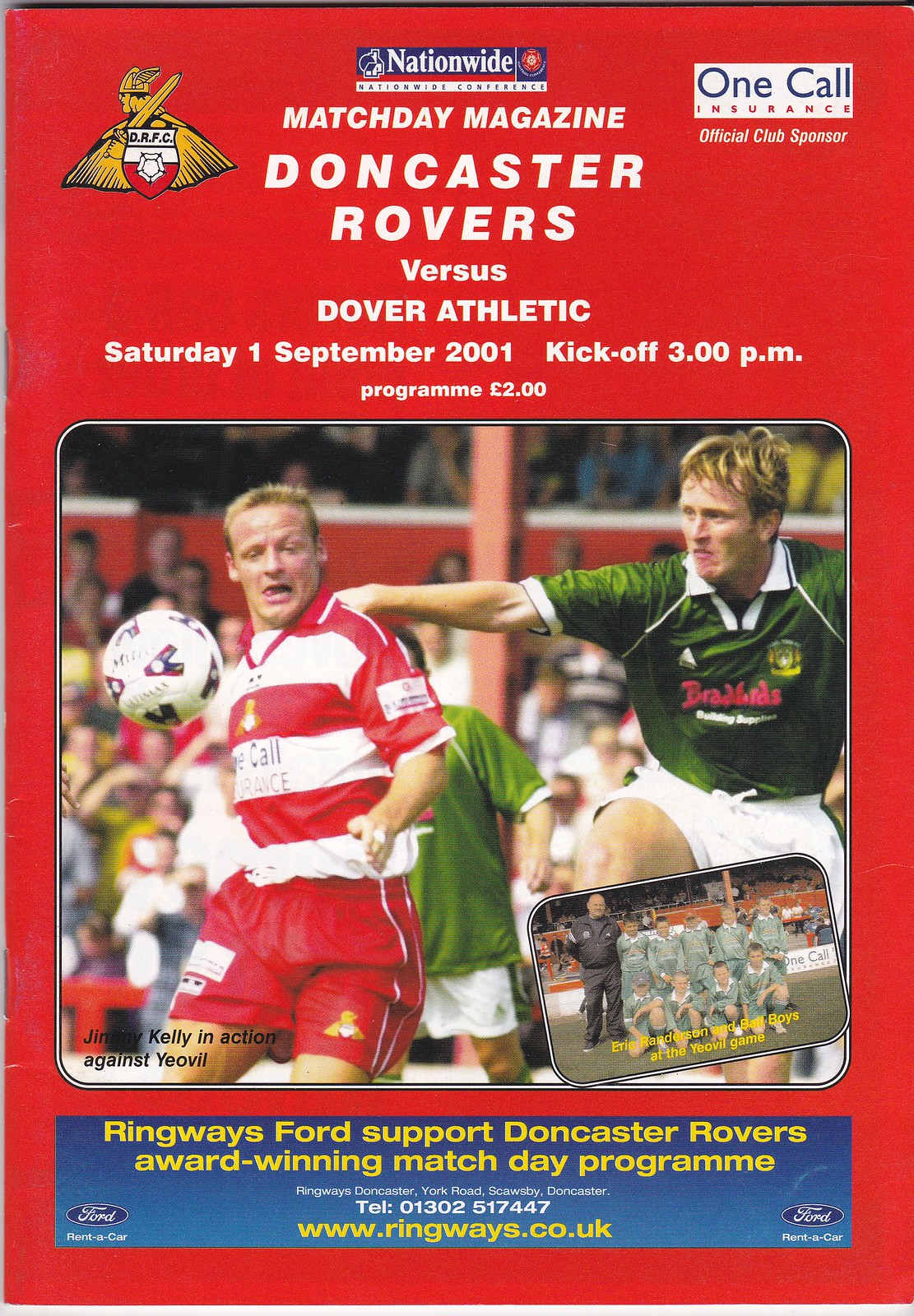The image is the cover of a Match Day Magazine for a soccer match between Doncaster Rovers and Dover Athletic, scheduled for Saturday, 1 September 2001, with a kickoff at 3 p.m. and the program priced at $2. The cover is predominantly red with white text at the top. In the center, there is a photograph of two soccer players competing for a ball midair, set against a backdrop of outdoor stadium stands filled with spectators. One player wears a red and white striped shirt with red shorts, while the other wears a green jersey with a white collar and white shorts. Several advertisements are scattered around the cover, including logos for One Call Insurance, Nationwide, and a football club symbol featuring a man with a sword and cape. In the bottom left corner of the photo, black text reads "Jimmy Kelly in action against UofL." Below the central image, a blue box with yellow text states, "Ringways Ford supports Doncaster Rovers award-winning Match Day program."